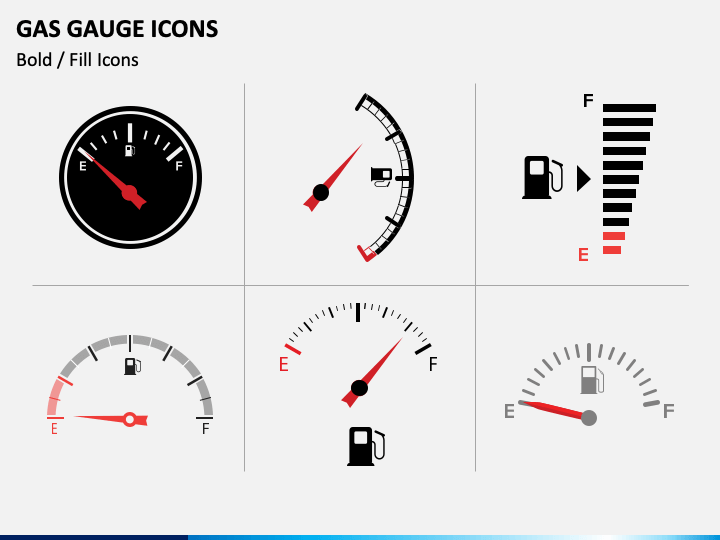This detailed graph presents various gas gauge icons under the title "Gas Gauge Icons: Bold/Fill Icons" located in the top left corner. The graph is organized into two rows, each comprising three distinct images.

**Top Row:**

1. **First Image:** A solid black circle contains a gas gauge. The letter 'E' is positioned on the left, a gas pump icon is in the center, and the letter 'F' is on the right, all in white lettering. The red needle points directly at 'E'.
2. **Second Image:** A curved line gas gauge shows a similar layout with 'E' on the left, a gas pump icon in the center, and 'F' on the right. Here, the red needle points upwards, indicating a higher fuel level.
3. **Third Image:** This gas gauge uses horizontal lines. A gas pump icon is on the left, accompanied by a series of horizontally aligned lines. Starting from the bottom, marked 'E' in red, two red lines gradually transition to longer lines, reaching the top where 'F' is indicated.

**Second Row:**

1. **Fourth Image:** Features a traditional curved gas gauge with 'E' on the left and 'F' on the right. In the center lies the gas pump icon, with the red needle positioned within the gauge.
2. **Fifth Image:** Exhibits a semicircular gas gauge where 'E' is on the left in red, 'F' is on the right, and the needle, also red, points close to 'F'. The gas pump icon is located underneath.
3. **Sixth Image:** Shows another semicircular gas gauge. 'E' is on the left (not colored red), 'F' is on the right, and the gas pump icon resides in the center while the red needle is positioned over 'E'.

The graph comprehensively illustrates the variations in gas gauge designs, from traditional to more abstract representations, highlighting their indicators and needle positions.